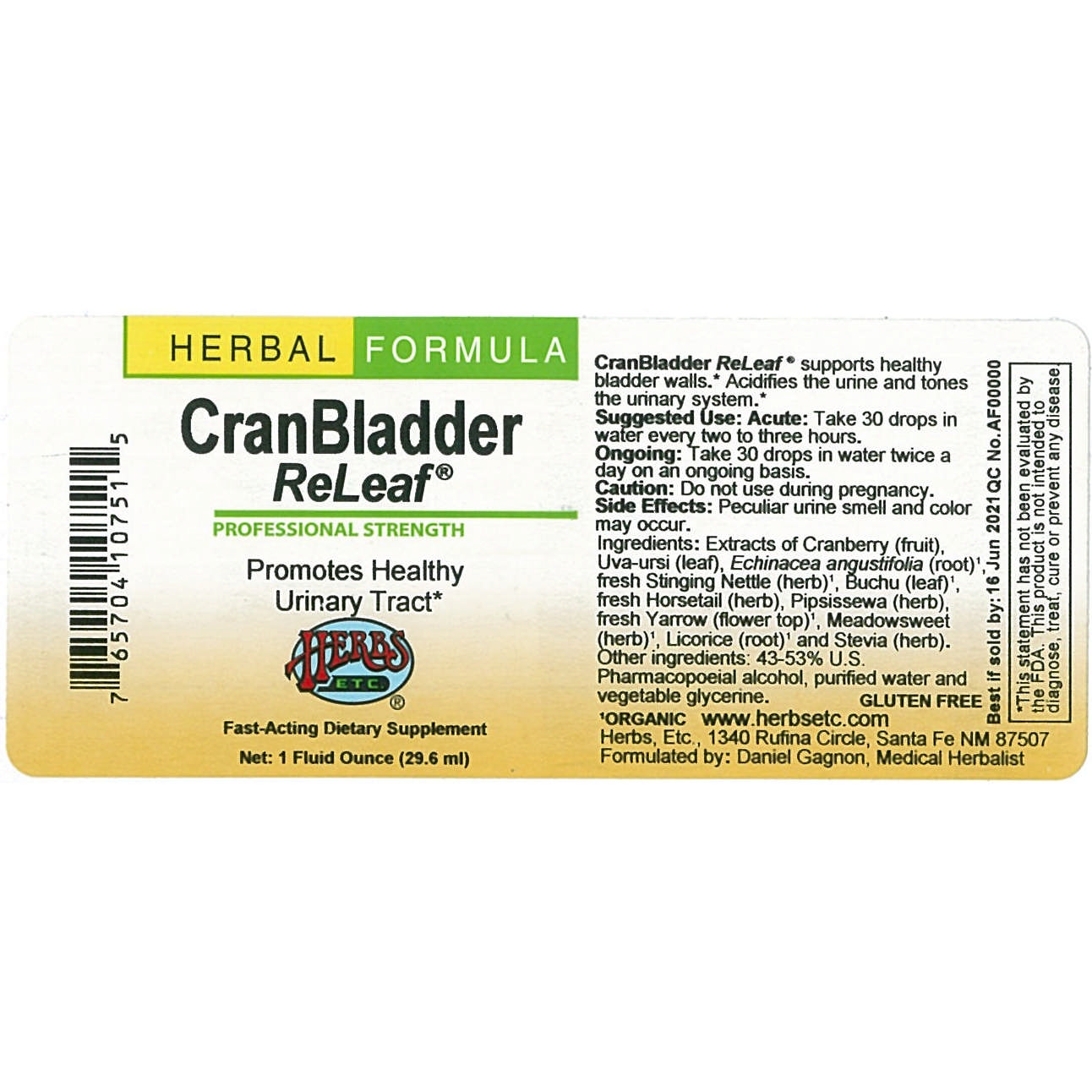This oblong label for a dietary supplement shifts from white at the top to a light golden yellow towards the bottom. On the far left side, it features a UPC code. The prominent section displays the product name "Herbal Formula, Cranbladder Relief (R-E-L-E-A-F)," indicating it is of professional strength and designed to promote a healthy urinary tract. The label identifies the manufacturer as "Herbs, etc." and describes the supplement as fast-acting. It includes specifications: Net 1 Fluid Ounce (29.6 milliliters).

The marketing section further elaborates that Cranbladder Relief supports healthy bladder walls, acidifies the urine, and tones the urinary system. For usage, it suggests taking 30 drops in water every 2-3 hours for acute conditions, and 30 drops in water twice a day for ongoing maintenance. 

The caution section advises against use during pregnancy. Possible side effects include a peculiar smell and color of urine. Ingredients start with cranberry extract, followed by Uva Ursi leaf and more, confirming that the product is gluten-free and organic. The provided website is www.herbsetc.com, and it lists their address. 

The far right side of the label features a "Best if sold by 16 June 2021" date, a QC number AF0000, and a disclaimer noting that the FDA has not evaluated the statements on the label, clarifying that the product is not intended to diagnose, treat, cure, or prevent any disease.